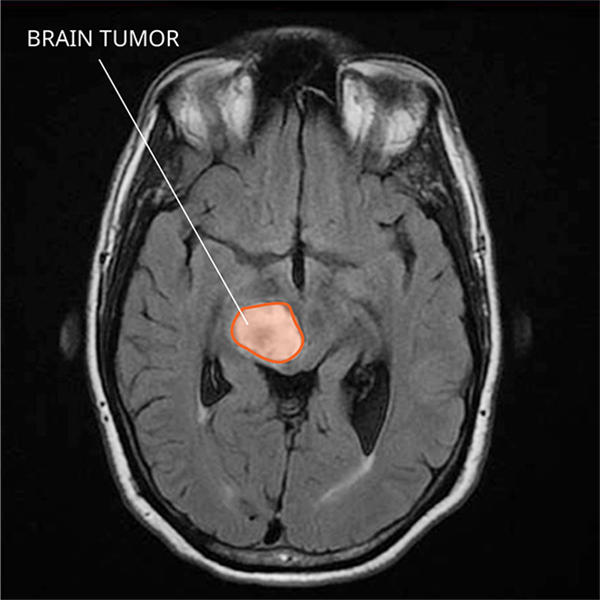The image is a black and white top-down view of a human brain, likely from an MRI or CT scan, with a dark background. The skull's outline is clearly visible, along with the eye sockets and the nasal cavity at the top of the image. Central to the brain is a highlighted area, marked with an orange or reddish-orange circle, presumably indicating a brain tumor. This portion is distinctly colored in a light pinkish or peach hue. A white arrow points from this circled region to the top left corner of the image, where the text "BRAIN TUMOR" is written in a thin, white font. The brain, rendered in varying shades of gray, contrasts sharply against the circled anomaly, emphasizing the abnormality for diagnostic reference.